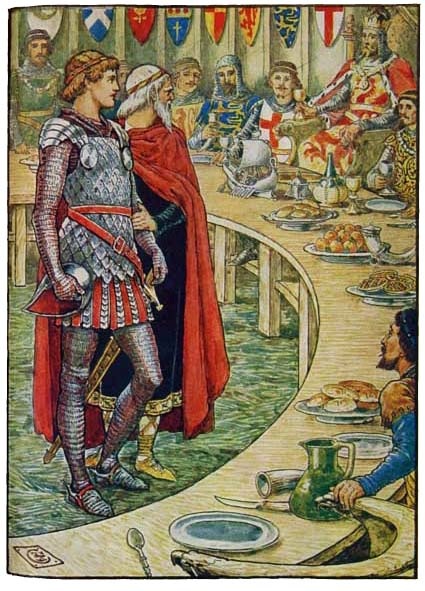The image, an exquisitely detailed classical painting, illustrates a grand dining room in a king's court, evocative of a medieval setting like those from the tales of King Arthur or Game of Thrones. Dominating the top right corner, the king is seated on his throne, adorned in a crown, a light tan tunic emblazoned with what might be a red dragon, and a rich red cloak. In the center of the scene stands a prince, armored in silver with a grey outfit, helmet, and a vibrant red cloak. Beside him, an older man with a beard, perhaps Merlin, wears a dark blue robe and a red shawl. The two are presented within the hollow of a grand round table, indicative of the legendary Round Table of Camelot. All around the table, which is a light brown wood color, men of Caucasian descent are seated, indulging in an array of food items that include round plates, jars, and drinks. The walls above are adorned with shields bearing various flags, adding to the medieval atmosphere. The scene, almost tarot card-like in its intricate and symbolic design, immerses the viewer in a storybook world of knights, kings, and grand feasts.